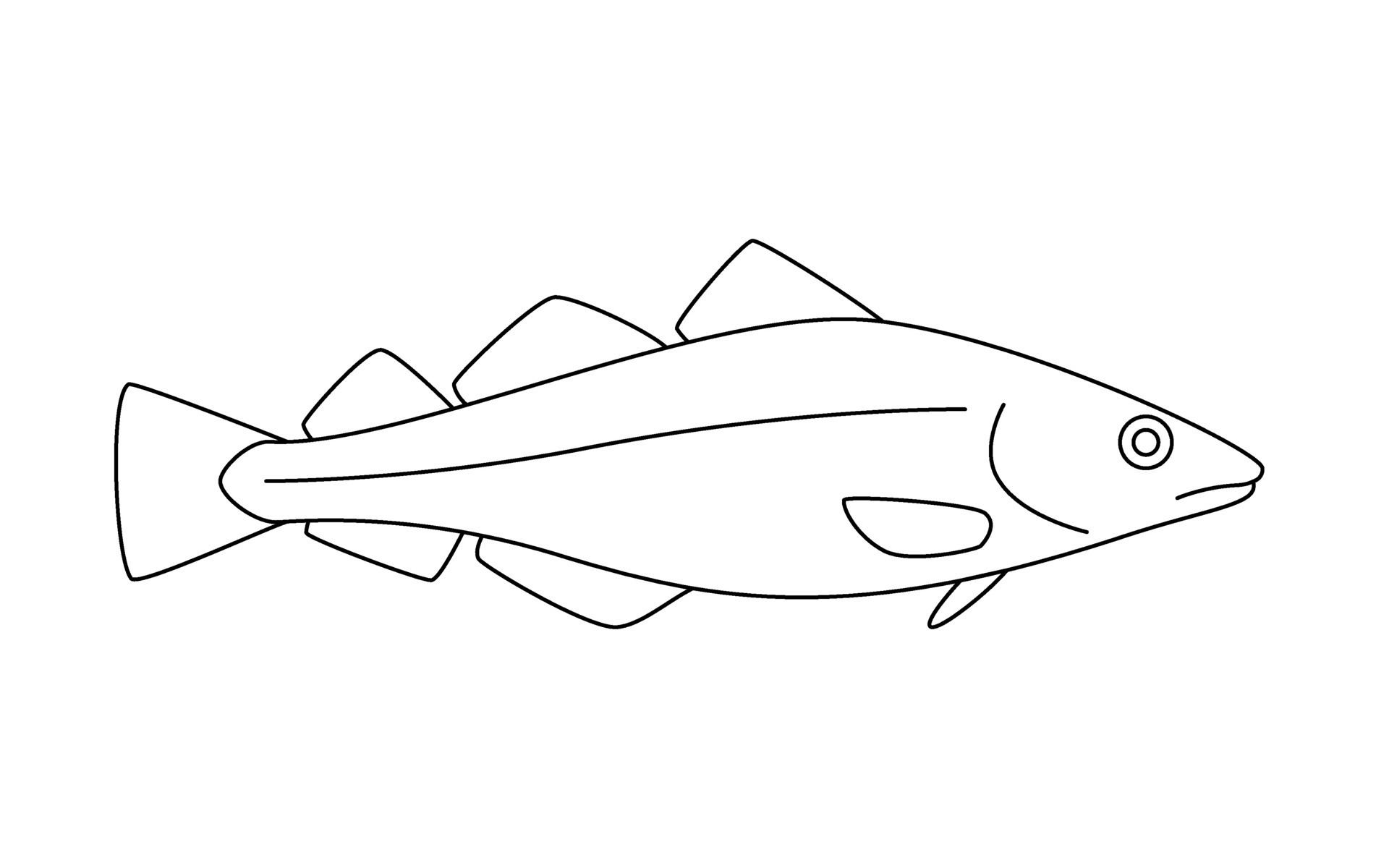The image features a line art sketch of a fish, oriented horizontally in the center against a plain white background. The fish is depicted in a side view with its tail end pointing towards the left and its nose towards the right. This graphical representation, likely computer-generated, uses black lines to outline the fish. It has a distinctively closed mouth and a circular eye, while the other eye is not visible due to the side view. The fish's body is characterized by three fins on the top and two on the bottom. Additionally, there are two more fins positioned near its head. A single curved line runs through the center of the fish, highlighting the anatomy further. Notably, no scales are depicted in the sketch, maintaining a simplified, clean aesthetic typical of line art style.